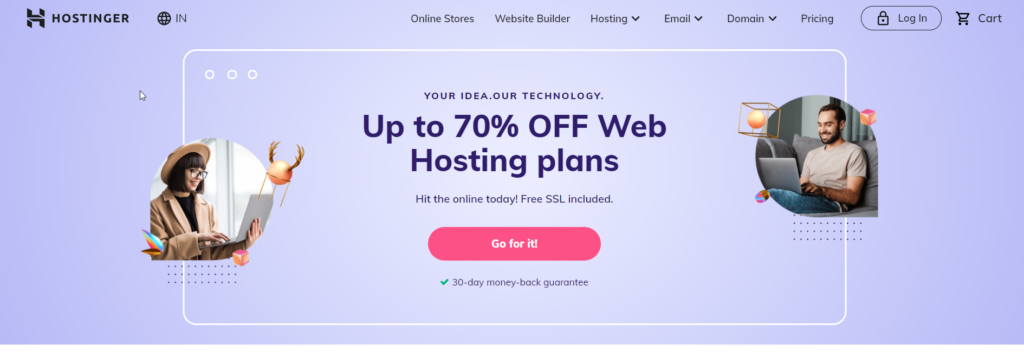The website interface features a light purple background with a subtle white sheen in the center, creating a gradient effect. In the upper left corner, a stylized "H" logo is displayed alongside the name "Hostinger" in bold, black, uppercase letters. To the right of this logo, there is a globe icon followed by the letters "IN".

Navigating towards the center of the page, the main menu options include "Online Stores", "Website Builder", "Hosting" (with a dropdown arrow for more options), "Email" (with a dropdown arrow for more options), "Domain" (with a dropdown arrow for more options), and "Pricing". Adjacent to these options is a "Login" button, accompanied by a lock icon and the word "Login". Moreover, a cart icon followed by the word "Cart" is visible at the far end of the menu.

Central to the page is a content window outlined in white, containing various elements. In the upper left corner of this window, three horizontally arranged circles can be seen. Below, there is an image of a smiling woman holding a gray laptop. She is dressed in a long tan coat over a black shirt, has dark brunette hair styled in a jaw-length bob, and wears glasses. She dons a round hat and holds a laptop from which whimsical character drawings emerge: a floating ball with deer antlers above the laptop, an orange cube below it, and a blue and orange abstract object to the left.

The center of the content window features the text "YOUR IDEA, OUR TECHNOLOGY" in uppercase purple letters, followed by “Continue” in purple text but in lowercase. Below this, it promotes "UP TO 70% OFF WEB HOSTING PLANS" with “OFF” in uppercase letters. The text "Hit the online today, free SSL included" appears directly underneath. A red button with white text labeled "Go for it" urges action, and a green checkmark followed by "30-day money-back guarantee" reinforces trust.

To the right, another circular image displays a smiling man using a laptop. He has short brunette hair and a beard, and he's dressed in a tan t-shirt and blue jeans. From his laptop emerge various whimsical graphics: an orange cube to the right, a brown transparent cube with an orange ball to the left, and a red and blue object below the laptop.